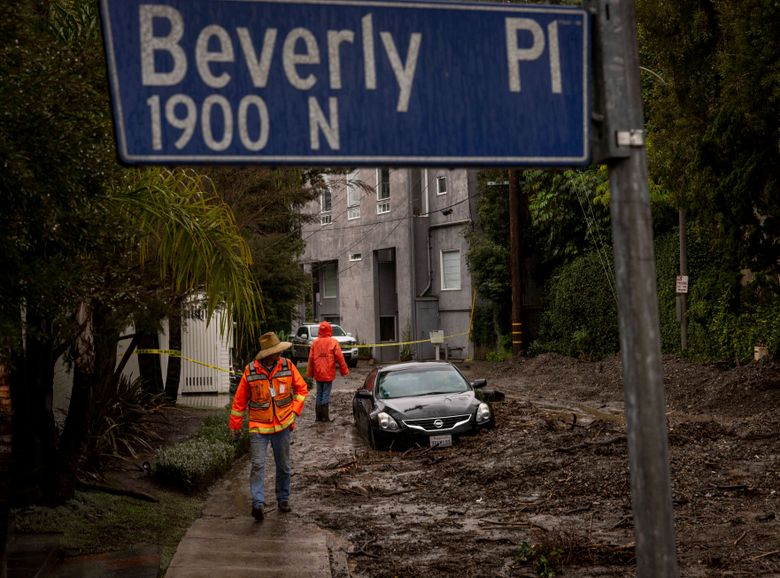The image captures the aftermath of a mudslide during daytime, vividly illustrating the extent of the damage. At the top of the photograph is a prominent blue street sign that reads "Beverly Place, 1900 North," supported by a steel pole. Below it, there's a multi-story apartment building made of gray stone or stucco. The street and sidewalks below are engulfed in mud, with the sidewalk partially visible and partially covered. Two men in orange safety jackets with jeans and boots are seen on the sidewalk - one walking towards the camera and the other moving away. In the street, a black sedan is submerged up to its license plate in the mud, immobilized. Vegetation, including palm trees and various other trees, frames the scene on both the left and right sides, their bases partially buried under the mud. The overall mood of the image conveys the chaos and disruption caused by the natural disaster.